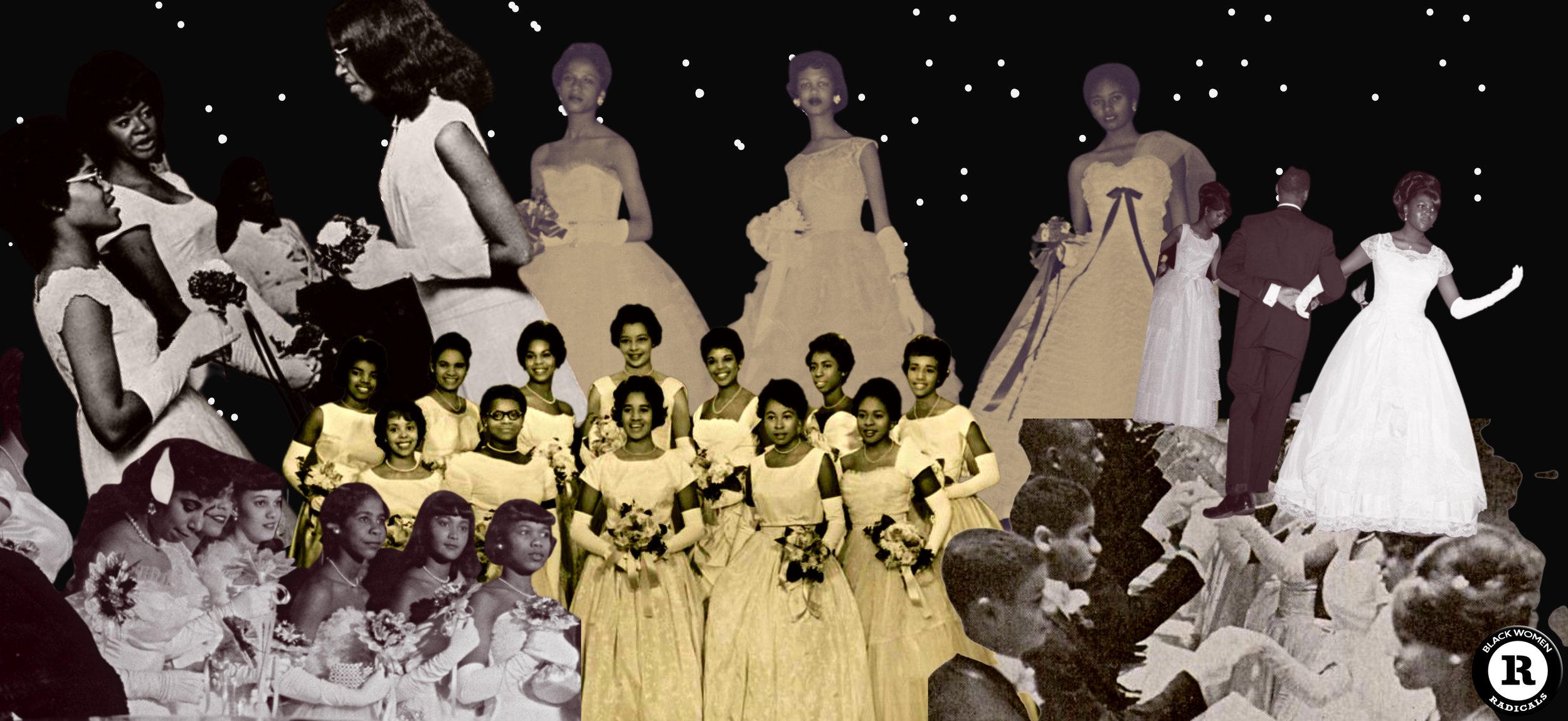The image is a detailed collage of photographs featuring African American women in formal white gowns, captured in various elegant settings. At the center, there's a notable large group photo where the women are dressed in long white dresses and gloves, each holding bouquets. Similarly, in the lower left, another group of women is seen in an identical formal attire. On the lower right, the collage depicts a lively ballroom scene where the women dance with men in tuxedos. The upper left section shows women in white gowns, holding bouquets and engaging in conversation. The collage also features the dynamic moment of a couple dancing on the right. Central to the top, three women in long white dresses pose confidently for the camera. The background of the collage is a deep black adorned with small white dots resembling stars, giving a celestial feel to the scene. On the lower right corner, the artwork is marked with the logo of Black Women Radicals, which features a capital letter 'R' in the center of a white circle, bordered in black. Overall, the collage harmonizes a diverse collection of black-and-white and warmer-toned images from different eras, united by the theme of celebration and elegance.